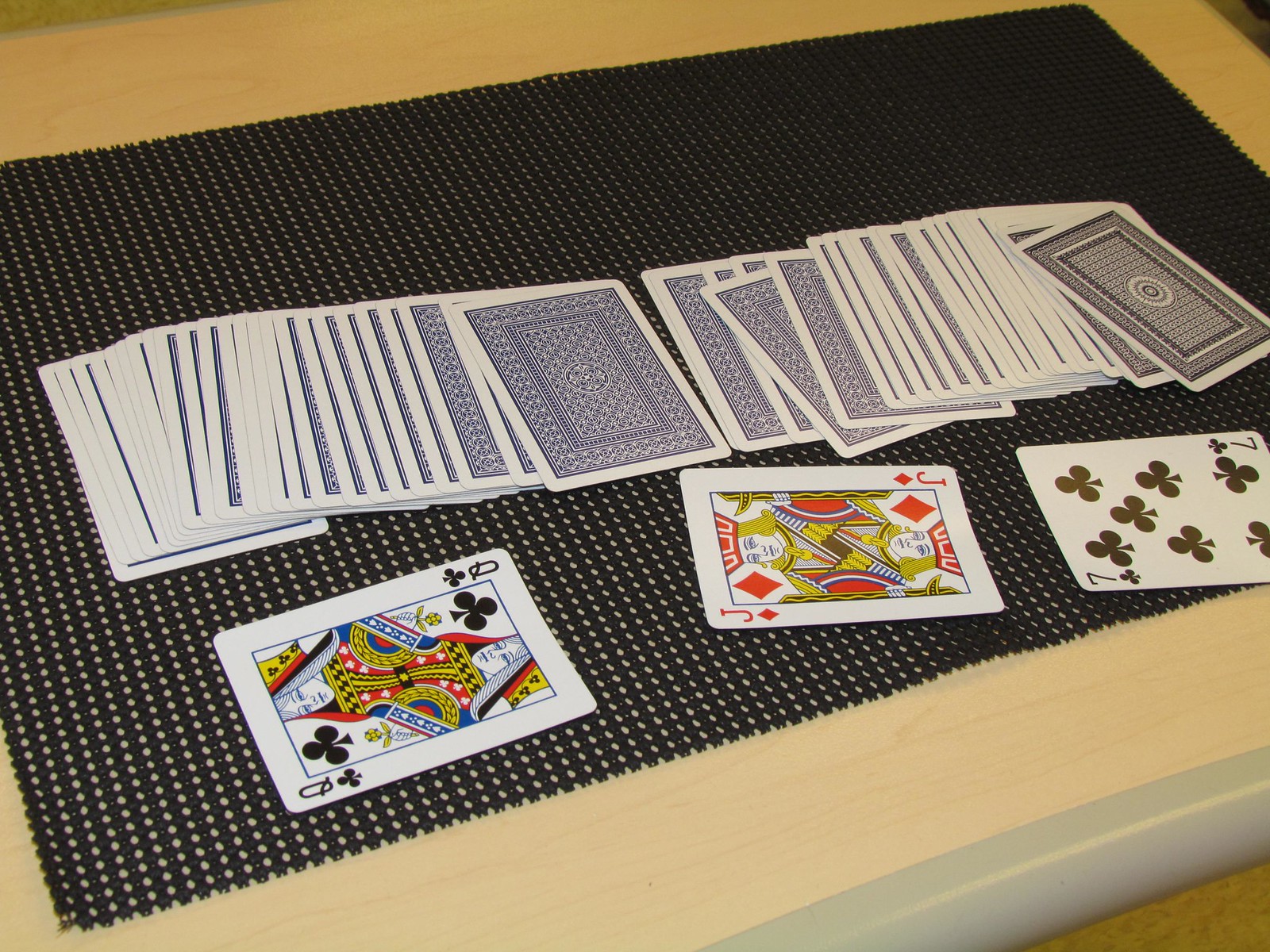The photograph captures a serene tabletop setting featuring a deck of cards intricately displayed. The table itself is a light tan hue with a distinctive gray border in the bottom right corner. Resting on this table is a black placemat adorned with white dots, presenting a tasteful contrast.

Prominently positioned across the center of the placemat is a deck of cards, exquisitely fanned out from left to right. The cards have a classic design with a white border encasing a blue patterned interior, each bearing a circle in the center. Notably, there appear to be two distinct decks, as observed by the cards on the far right side which are a darker blue with a different focal design.

Adding to the composition, a queen of clubs card is laid horizontally at the bottom left of the fanned array, while a jack of diamonds is similarly placed to its immediate right. Towards the far right corner, the image captures a seven of clubs card that partially extends off the placemat, with the camera cutting off the bottom right corner of the card, rendering it incomplete in the frame. This meticulous arrangement creates a visually engaging and detailed depiction of a classic game in progress.